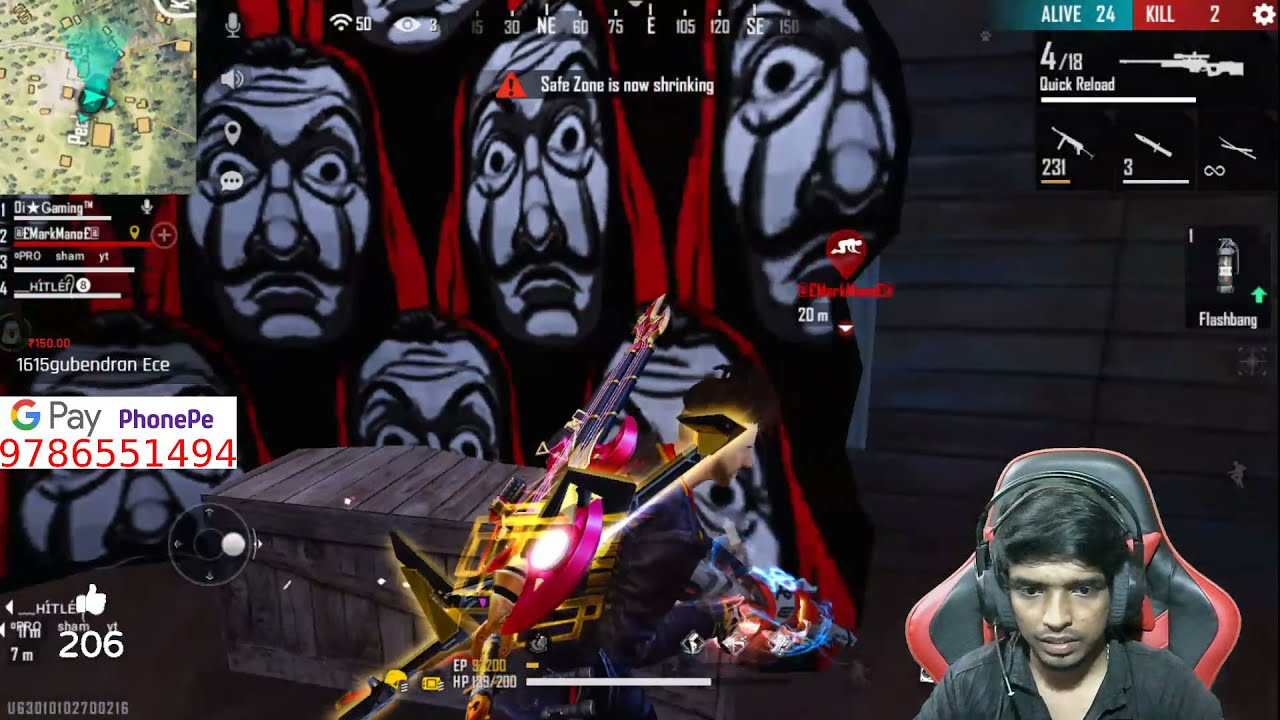The image is a detailed screenshot from a video game stream. In the bottom right corner, there’s a picture-in-picture view of the streamer - a man with dark brown skin, black hair, and a black shirt, seated in a high-back gaming chair with a black cushion outlined in red. He’s wearing a black headset with a microphone in front of his face.

The center of the image displays the player's character in the game, armed and amidst action. To the upper right, there's a scoreboard: green text indicates "live 24", red text reads "kill 2", and beneath them is a gear icon with "4/18 quick reload" in white text, accompanied by an arrow pointing left.

A horizontal bar appears below these indicators, followed by images of weapons: a rifle with "231" underneath, a knife with "3", and a lamp labeled "flashbang" with a green upward arrow. An illuminated guitar with two necks and a bright light at its center is prominent in the game's visuals, surrounded by the faces of several men with wide eyes, gray skin, black facial lines, and red scarves.

The top center showcases a complex gauge marked with various values and codes, while a gray line with a red triangle and exclamation mark below warns, "safe zone is now shrinking".

In the far upper left corner, there’s a game map. Underneath it is a scoreboard listing the top four players by name. Beneath this are several icons and text: a white box with the Google Pay symbol and "Phone PE", followed by the number "9786551494", and finally "206" with a thumbs up emoji above it, suggesting viewer interactions, possibly for tipping the streamer.

The entire scene is vibrant with various colors: the streamer’s interface and game elements merge greys, reds, blacks, and other hues, depicting a lively and dynamic atmosphere within the video game.